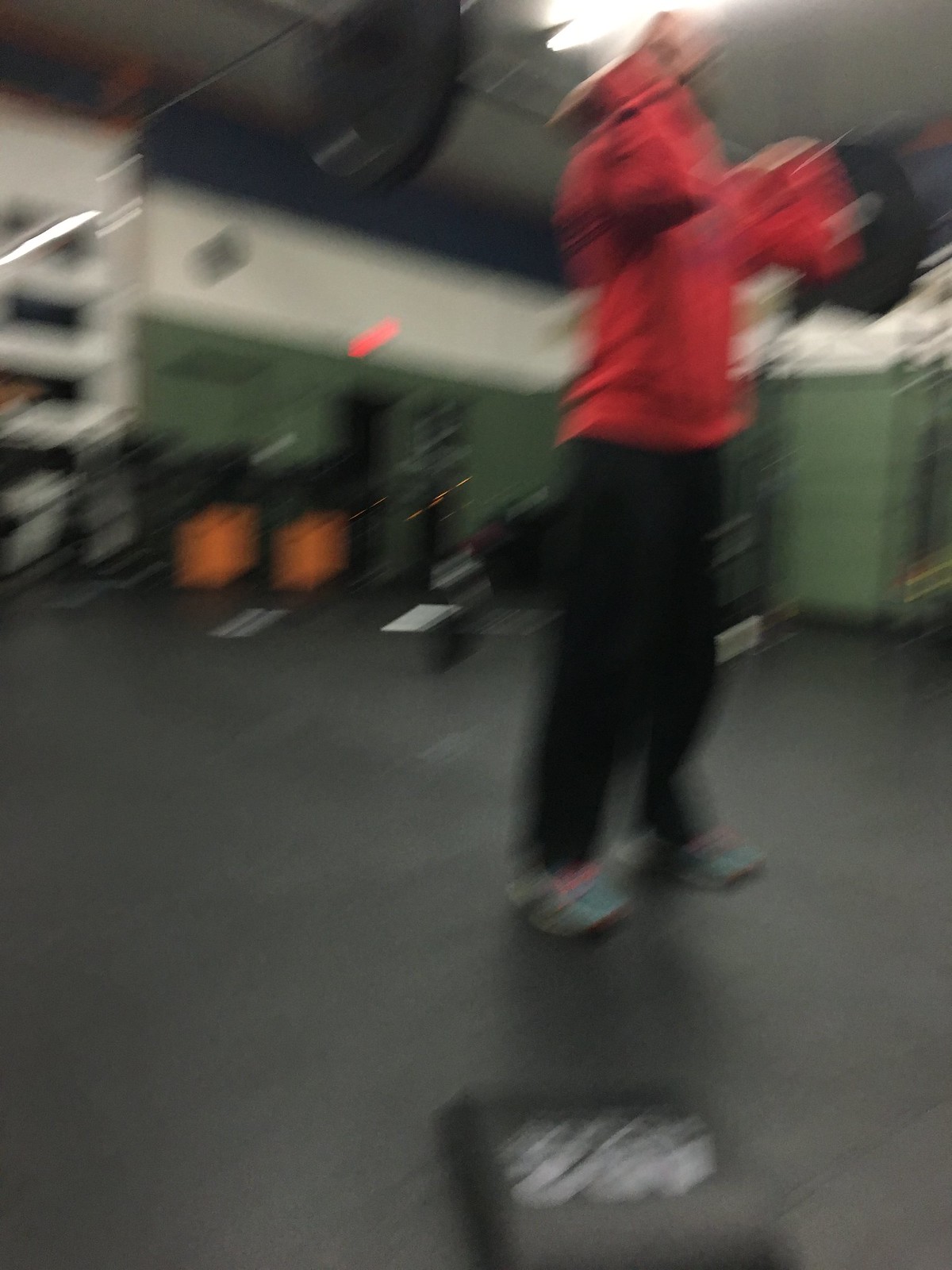In the image, there is a heavily blurred background featuring shades of brown and gray, with indistinct shapes suggesting the ground. A person stands at the center of the image, preparing to do squats. He is holding a metal barbell across his shoulders, which is weighted on both sides. The individual is wearing a baseball cap backward, which appears to be white, along with a red sweater. He is also dressed in black pants and sneakers. 

In the background, there is a light, possibly a stripe, visible at the top and some green hues near the bottom. There seem to be various equipment and shelves, perhaps holding electronics or workout gear, though these elements are quite out of focus. The left side of the background particularly features more shelves and a noticeable white light, amidst an overarching grayish tone.